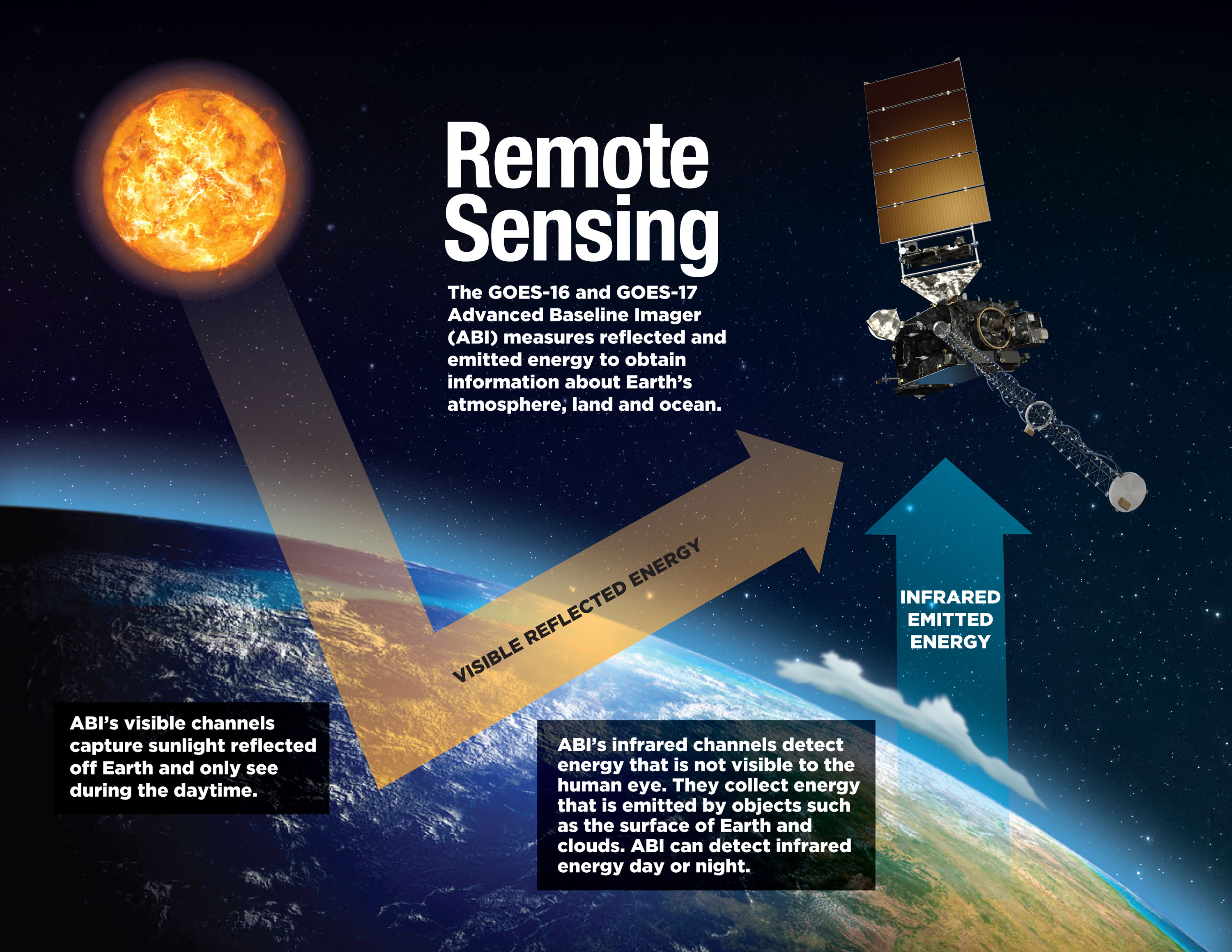This well-designed infographic illustrates the relationship between the Sun, the Earth, and a satellite within a dark bluish-black gradient space filled with stars. The Earth occupies most of the bottom of the graphic, showcasing green and brown land with blue oceans and possibly clouds or mountains. The Sun, shown glowing with shades of orange, red, and yellow, is positioned at the top left. The satellite, featuring copper-colored solar panels and elements of gold, white, and black, is situated at the top right.

In the top center, large white text reads "Remote Sensing," followed by a detailed description in smaller white text: "The GOES-16 and GOES-17 Advanced Baseline Imager (ABI) measures reflected and emitted energy to obtain information about Earth's atmosphere, land, and ocean."

A semi-transparent orange arrow extends from the Sun, makes a 90-degree turn on reaching the Earth's surface, and points towards the satellite. Inside this arrow, black text reads "Visible reflected energy." Another semi-transparent light blue arrow originates from the Earth and points upwards towards the satellite with white text inside that reads "Infrared emitted energy."

Additional explanatory text is provided in white on black backgrounds. In the bottom left corner, it reads: "ABI's visible channels capture sunlight reflected off Earth and only see during the daytime." On the right side of the Earth, it states: "ABI's infrared channels detect energy that is not visible to the human eye. They collect energy emitted by objects such as the surface of Earth and clouds. ABI can detect infrared energy day or night."

Overall, the infographic provides a comprehensive and visually engaging representation of how the ABI on the GOES-16 and GOES-17 satellites measures reflected and emitted energy to gather detailed information about Earth's atmospheric, terrestrial, and oceanic conditions.